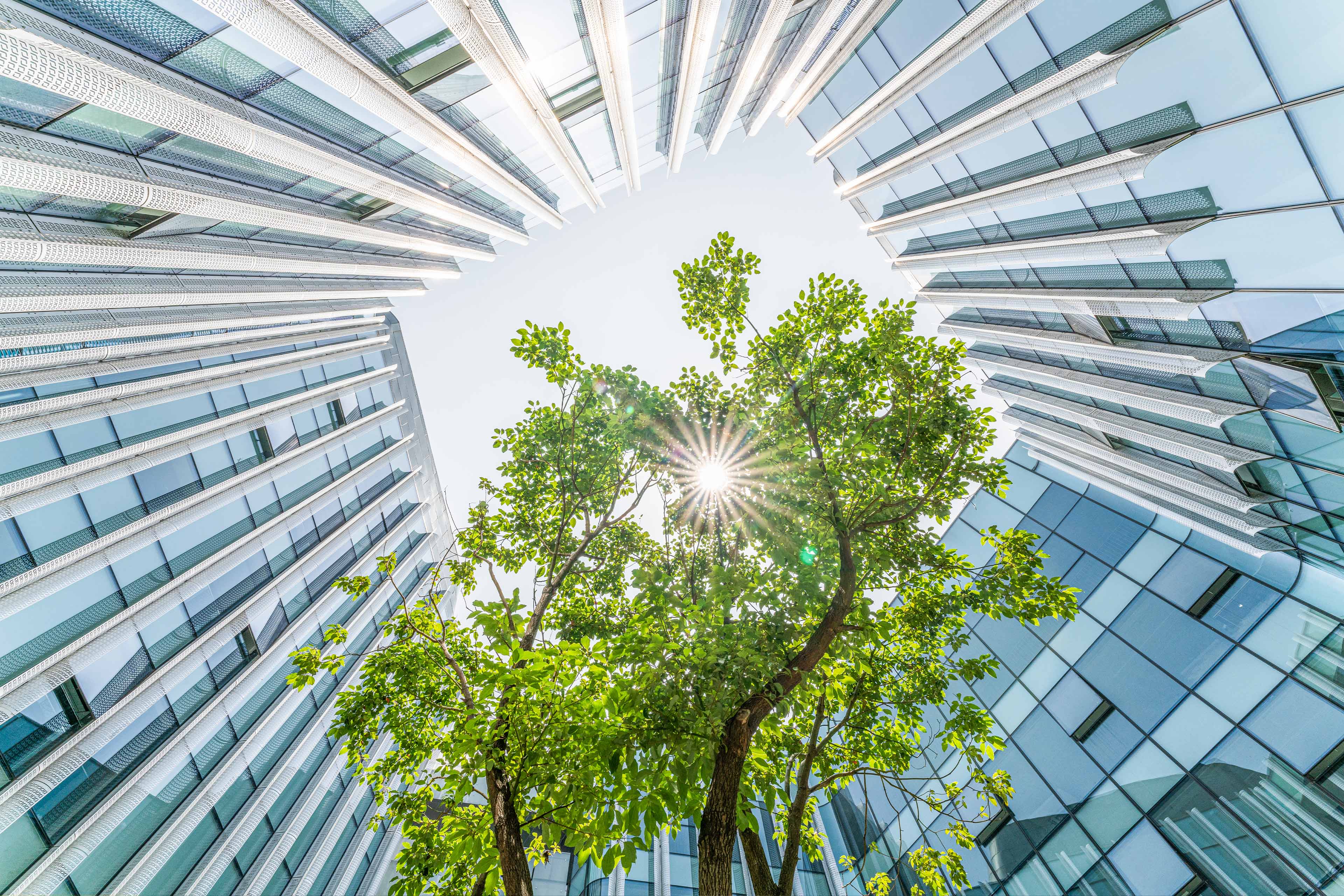The image captures an upward perspective from the bottom of a modern courtyard encircled by towering, reflective glass skyscrapers. Each side of the frame showcases the sleek, blue-tinted windows of these buildings, creating a sense of being enclosed by urban architecture. In the center of this contemporary courtyard stands a tall, vibrant tree with lush, green leaves. The tree partially obscures the sun, allowing sun rays to filter through its branches and leaves, casting a gentle glow across the scene. The sky above appears light and slightly whitish, contrasting with the polished glass facades of the surrounding structures, which reflect the serene atmosphere of a sunny day.